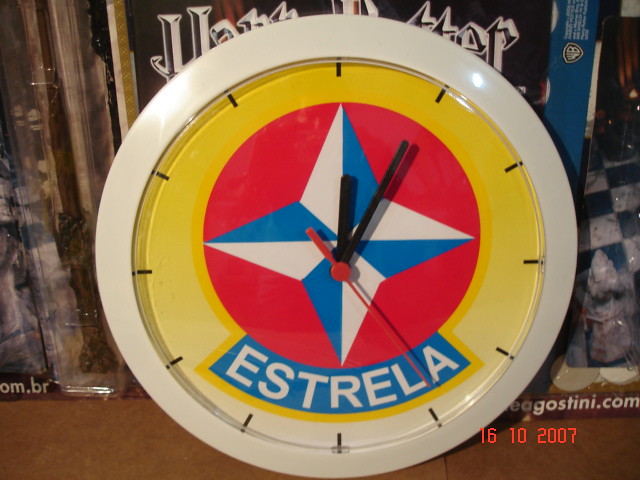This image showcases a distinctive clock with a white outer edge encased in a clear bezel. The clock face features a vibrant design with a yellow inner ring and a red center. A blue and white-shaded star with four points is prominently displayed in the center. The word "Australia" is inscribed in white letters against a blue background. The clock does not have traditional numbered markings; instead, hours are indicated by simple lines. The time on the clock reads approximately 12:05, with both the hour and minute hands visible. 

In the background, there is a Harry Potter-themed item, which could be either a glass ornament or a book, providing a whimsical backdrop to the clock. At the bottom of the image, a date stamp reads "16-10-2007," suggesting when the photo was taken or the item was made. Additional text in the background includes the partially visible web address "e-a-g-o-s-t-i-n-i.com," hinting at a source or manufacturer of the product. The overall composition of the photo brings together elements of timekeeping, cultural reference, and themed merchandise.